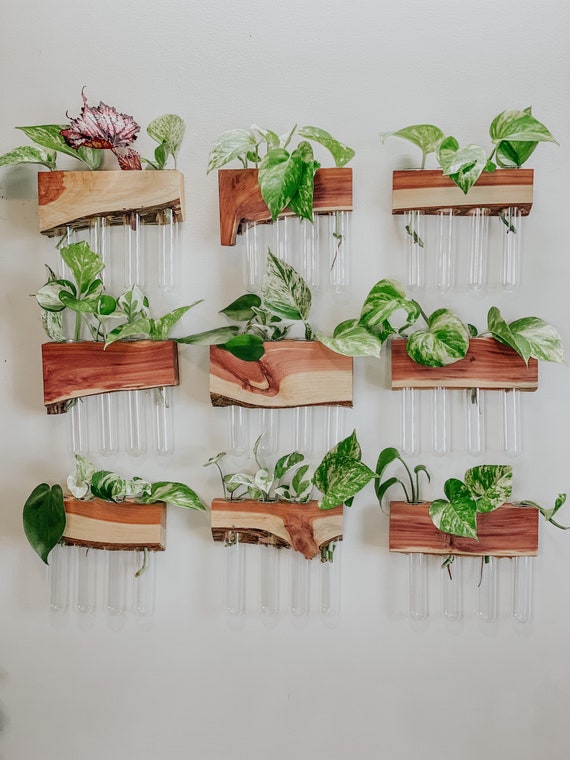The image displays a soft gray background with nine wooden wall-mounted blocks, arranged in a grid of three rows and three columns. Each wooden block is unique, showcasing different textures and designs, some resembling redwood with red and white streaks. Each block has holes drilled at the top, from which four clear glass or plastic test tubes hang. The test tubes are filled with various plants, their green leaves cascading out and some roots visible through the clear containers. One notable plant in the top left block appears wilted, with white and dark red colors contrasting against the predominantly green leaves of the other healthy plants. This wall-mounted garden setup creates a visually striking home garden.